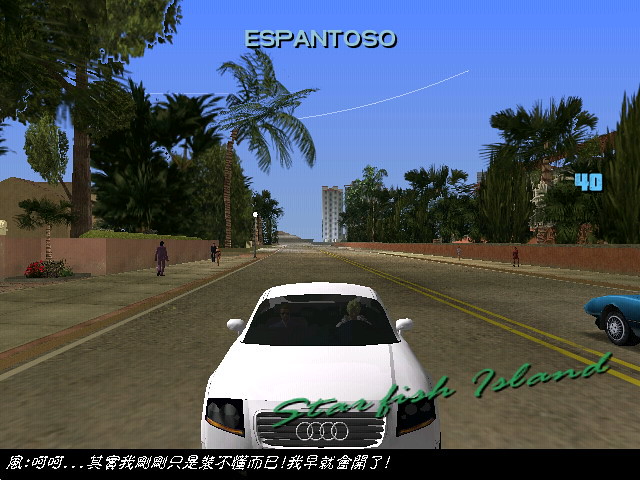This image appears to be a rendering from a video game, depicting a sunlit street scene under a vivid blue sky. A streak in the sky suggests a jet passing by, leaving a light gray trail. Dominating the background is a tall, gray building at the end of a two-lane road, marked by a double yellow line running down its center. The road is flanked by sidewalks lined with towering palm trees and other tropical vegetation.

In the distance on the left-hand side of the road, two figures are seen walking, while a single figure walks on the right-hand side. Prominently featured in the foreground, a white Audi car faces the viewer, identifiable by its signature grill with four interlocking silver rings. The car appears to have a driver inside.

Additionally, a blue car is partially visible on the right edge of the image, traveling in the opposite direction. The scene includes text elements, with "ESPANTOSO" displayed at the top, suggesting a Spanish influence, and "Starfish Island" written in green cursive at the bottom right. Below this, there is a black bar with white characters, possibly in Japanese or Chinese. The number 40 is noted in light blue on the right side of the image, completing the detailed depiction.